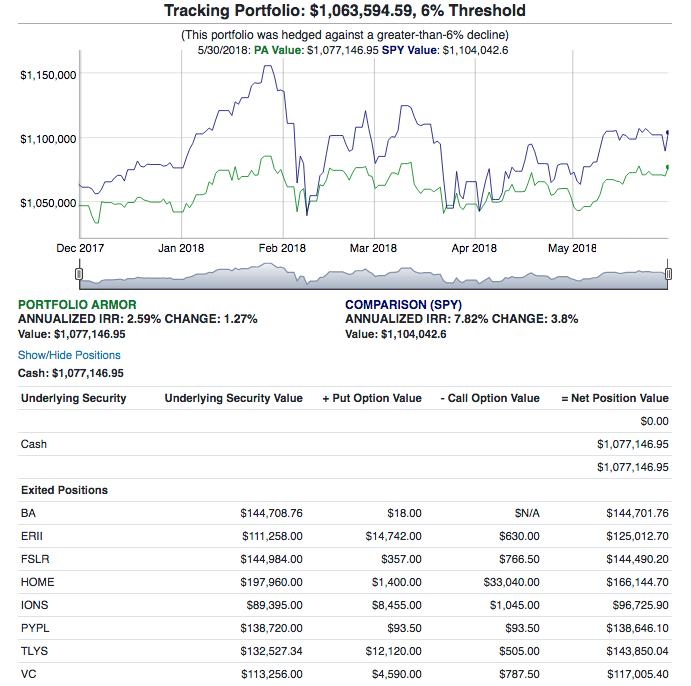This image depicts a detailed tracking portfolio on a clean white background. At the top center, the title "Tracking Portfolio" is displayed, along with the current portfolio value of $1,063,594.59 and a 6% threshold. A gray line separates this header from the main content below.

Prominently featured is a large rectangular line graph. Above the graph, a note indicates that the portfolio is hedged against declines greater than 6%. The graph is dated "5-30-2018" and showcases two prominent values: the PA value in green at $1,077,146.95 and the SPY value in blue at $1,104,042.06. The graph itself is color-coded, with green and blue lines representing the PA and SPY values, respectively. The left side of the graph is marked with numerical values, and the bottom is lined with dates.

Below the graph, additional portfolio details are provided. On the left side, the label "Portfolio Armor" is highlighted in green, indicating an annualized IRR of 2.59% and a change of 1.27. To the right, under the heading "Comparison (SPY)," it lists the cash value as $1,077,146.95. Further below, columns detail the following categories: "Underlying Security," "Underlying Security Value," "Put Option Value," "Call Option Value," and "Net Position Value."